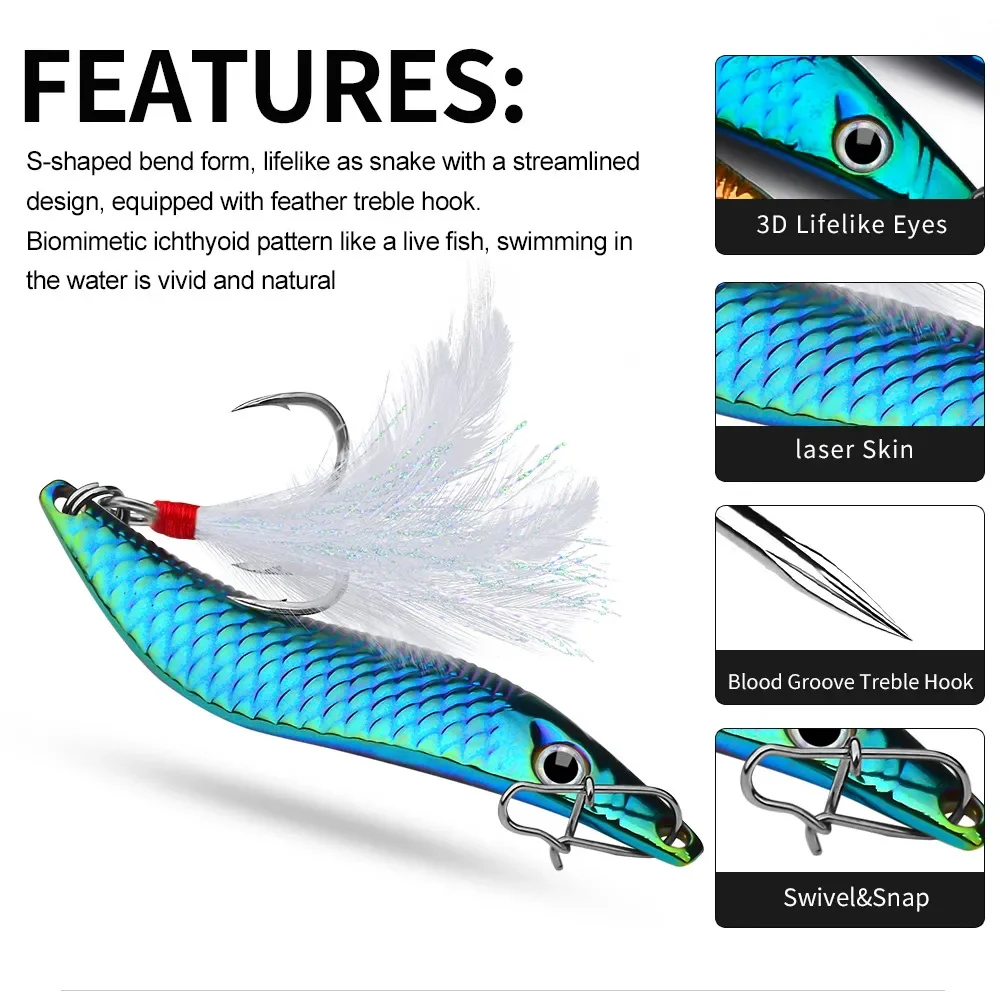Features: An F-shaped bend form designed to be lifelike with a streamlined structure and equipped with a feathered treble hook. It showcases a biomimetic, archified thyroid pattern that vividly imitates the natural swimming motion of a live fish. The fishing lure displays a vivid blue coloration with some green scales, enhanced by an iridescent sheen. The design includes 3D lifelike eyes, a laser-etched skin, and a blood groove treble hook, providing a realistic and natural appearance. The lure's mouth features a hole housing another metal hood or clasp, and a white feather accentuates the treble hook at the rear. The top right corner features additional details such as "3D lifelike eyes, laser skin, blood groove, treble hook, and swivel and snap." The product is set against a clean, white background with bold black text highlighting its impressive features.